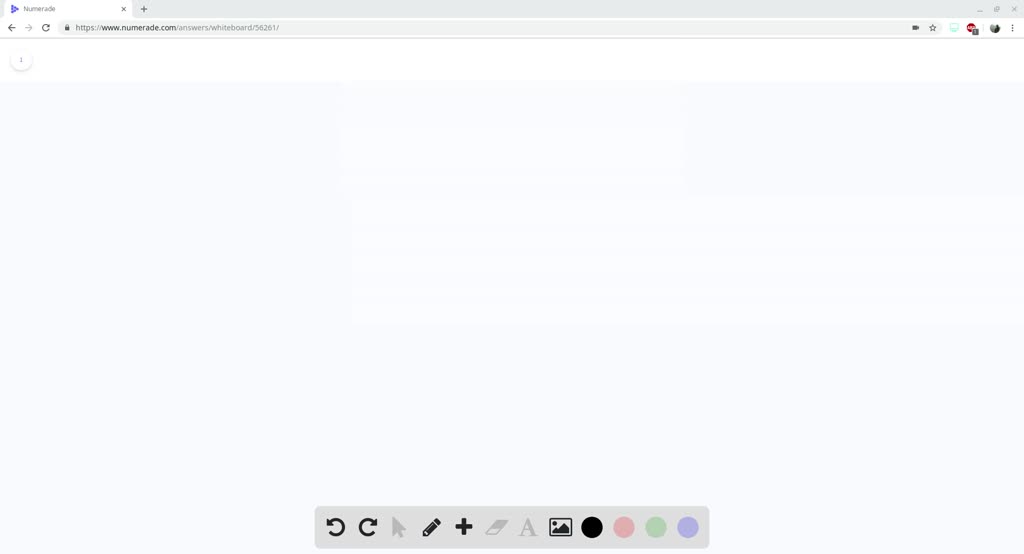Caption: "The image showcases a screenshot from a website, visible on someone’s computer screen. The URL bar at the top reads 'www.numeraid.com,' although the text is slightly unclear. The main body of the webpage features a large, light blue rectangle occupying the center, which appears to be a blank canvas. At the bottom of the page, there is a gray toolbar with various icons designed for interactive drawing. These icons include a return arrow, backward and forward arrows, a plain arrow, a pencil, a plus sign, an eraser, an 'A', an image icon, and four colored circles in black, pink, green, and purple, presumably indicating color choices for drawing."